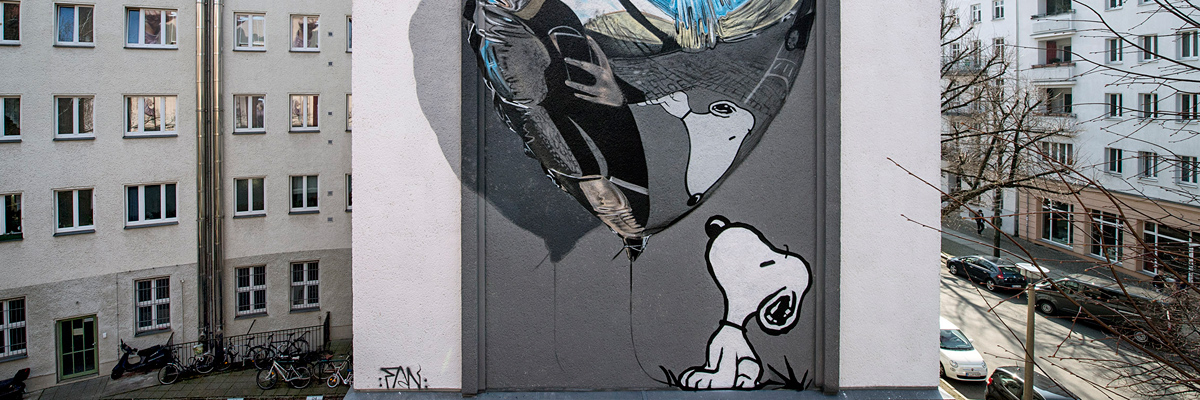This detailed photograph captures street art painted on the side of a building at rooftop level, likely on the doors of an elevator shaft. The central artwork features Snoopy the dog on a gray background, gazing up at his reflection in a foil heart-shaped balloon above him. A hand holding a cell phone is also visible in the balloon's reflection. The wall with Snoopy's painting is flanked by white strips and positioned between two multi-story buildings, one on the left with a bike rack containing four bikes at the bottom, and another on the right. In the broader context, the image reveals a street scene with leafless trees—suggesting fall—and several cars parked on the right side.